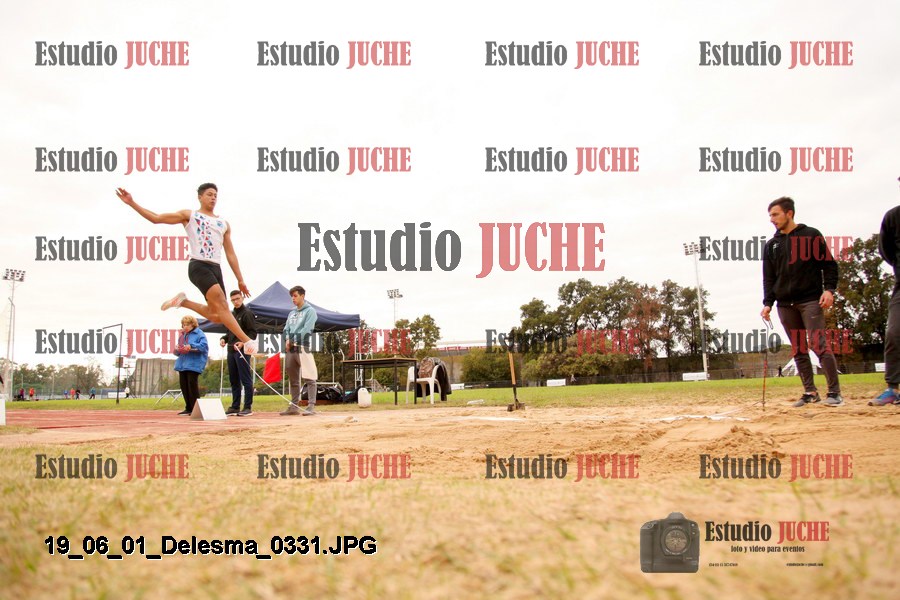This image captures a dynamic moment at a track event, set against a field with patches of dirt and grass. Prominently overlaid on the picture are the words "The Studio Juche," with "Studio" in black and "Juche" in red text. This superimposed text repeats in various lines across the image, suggesting it might be an advertisement or promotional material. In the bottom right corner, near a small camera icon, the words "Estudio Juice" appear again, likely indicating the name or brand involved.

The focal point of the image is a track athlete in mid-air, performing what seems to be a long jump. The athlete is clad in a white sleeveless shirt, black bike shorts, and white cleats. Their left leg is bent back from the knee, while the right leg extends forward in an elegant arc. Off to the left, a dark blue canopy tent shelters three onlookers, who appear to be observing the athlete's performance. There is also another man situated in the right center of the image, dressed in a black sweatshirt, gray pants, and tennis shoes, attentively watching the jumper.

The background provides a verdant contrast, showcasing grass and trees that frame the scene. An additional detail at the bottom left corner of the image reads "19-06-01-delezma-0331.jpg," likely indicating the file name or a timestamp for the photograph. The image's composition and the elements captured within it vividly convey the intensity and energy of the track event.